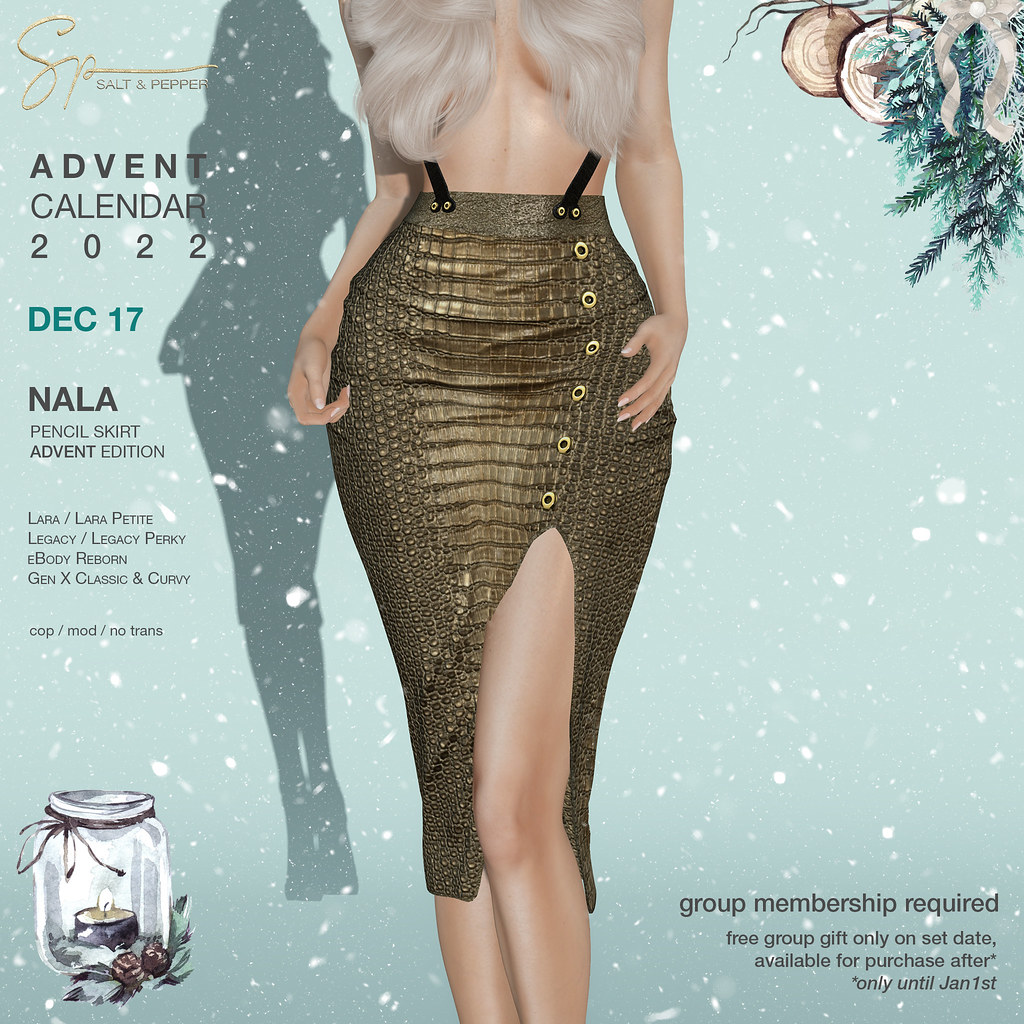The image is a detailed advertisement for a pencil skirt featured in an Advent Calendar 2022 edition. The central focus is a woman shown from her shoulders down to her calves. She is wearing a dark copper, alligator-skin pattern pencil skirt with gold embellishments. Her chest is covered by her long, gray hair. Black strings, resembling suspenders, go up towards her shoulders, while her arms hang down naturally with her hands by her hips. To the right of her skirt, metal buttons run down to an opening where her leg is visible.

In the top left corner, gold cursive letters spell out "SP," followed by "Salt and Pepper." Below this, in black letters, are "Advent Calendar 2022" and "December 17." Further descriptions detail the skirt's features, noting it as a "pencil skirt, Advent edition," compatible with various body types like Lara, Legacy, eBody Reborn, and Gen X Classic and Curvy. The terms "cop / mod / no trans" are also mentioned.

The upper right corner includes festive decorations with green pine branches, two wood slice ornaments, and a white ribbon. Below, on the bottom left corner, is an illustration of a mason jar with a lit candle, adorned with greenery. The light green background is speckled with white, resembling snowfall, and the figure casts a shadow on the left side of the background.

In the bottom right corner, text mentions "group membership required, free group gift only on set date, available for purchase after only until January 1st." The overall aesthetic is festive and detailed, emphasizing the exclusivity and seasonal theme of the product.